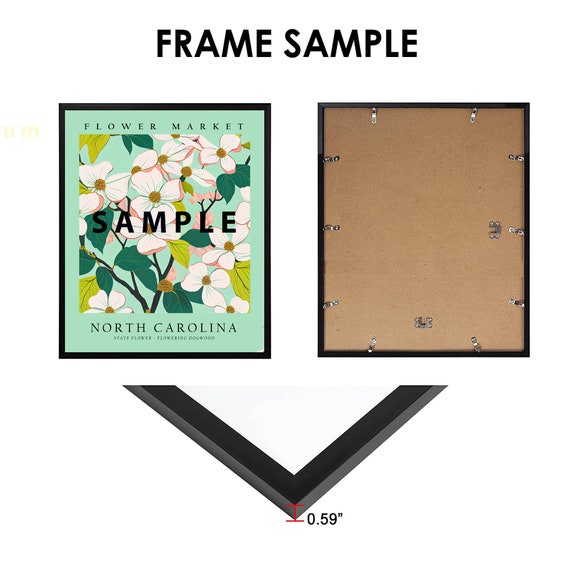This image displays a detailed sample of a picture frame advertisement. At the top of the vertical image, "Frame Sample" is prominently featured in bold black letters. The image includes two distinct parts: 

On the left, a black frame encloses a vibrant picture depicting white flowers with yellow centers and surrounding green leaves. The picture label reads "Flower Market" at the top and "North Carolina" beneath it. Centrally, the word "Sample" is boldly overlaid across the floral image.

On the right, a view of the back of the frame is shown, highlighting its brown cardboard backing and securing black edges. The back displays the metallic clips used for holding the picture in place. Additionally, a black V-shaped symbol with a line extending from its point is located at the bottom. This line has a small label next to it, indicating a measurement of "0.59 inch," which likely refers to the frame's internal spacing or border width.

This comprehensive display not only exemplifies the frame's design and functional aspects but also highlights its decorative potential with floral art.